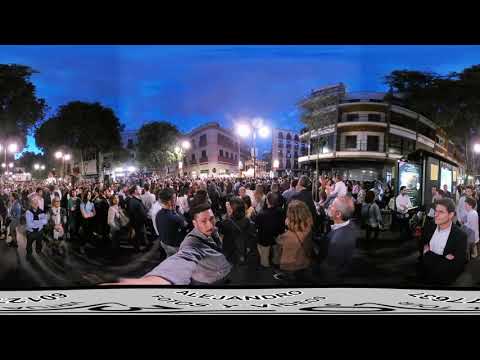The image captures a vibrant street scene just as evening settles in, with the sky a deep, dusky blue partially covered by clouds. The area is bathed in the warm glow of multiple streetlights, each mounted on black posts with three large lamps illuminating the area. A man, dressed in a gray long-sleeve button-up shirt and wearing a black crossbody bag, takes a selfie with a 360-degree camera, evident from the image's warped perspective and his elongated arm. Behind him, a sizeable crowd—likely hundreds of people—is congregating, filling the street in what appears to be a festive or bustling urban setting, reminiscent of places like Bourbon Street in New Orleans. On the right side of the image stands a four-story apartment building with balconies and a black bus shelter adorned with advertisements. The buildings are a mix of light gray and light pink hues, adding to the scene’s visual interest. Interspersed among these structures are healthy, green-leaved trees contributing to the lively and dynamic skyline.